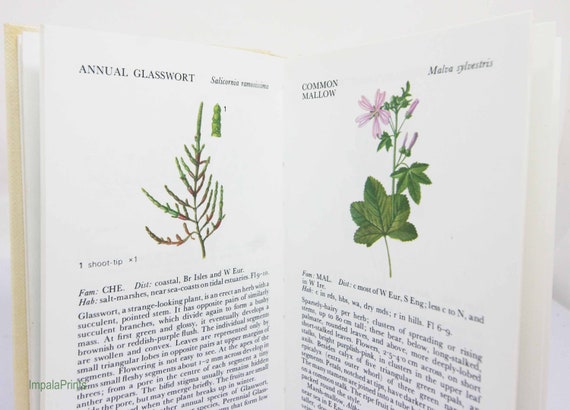In a square, full-color indoor photograph illuminated by artificial light, an open hardcover book with a light brown cover occupies the center against a primarily white background. The book reveals two pages featuring botanical illustrations and descriptions. 

The left page presents an illustration of a plant identified as "Annual Glasswort" at the top-left corner, with further scientific details below that are too small to read clearly. This plant has a spiny, succulent stem, described as an erect herb. The illustration suggests a fern-like appearance with greenish leaves.

The right page showcases another botanical drawing of a "Common Mallow" at the top-left corner, with the scientific name "Malva sylvestris" possibly listed at the top-right. This plant is depicted with large green leaves, pink flowers, and pinkish-purple buds at various stages of blooming. Additional text beneath the illustration includes a brief scientific description followed by paragraphs of detailed information about the plant's characteristics, which mentions clusters of spreading or rising stems up to 80 centimeters tall.